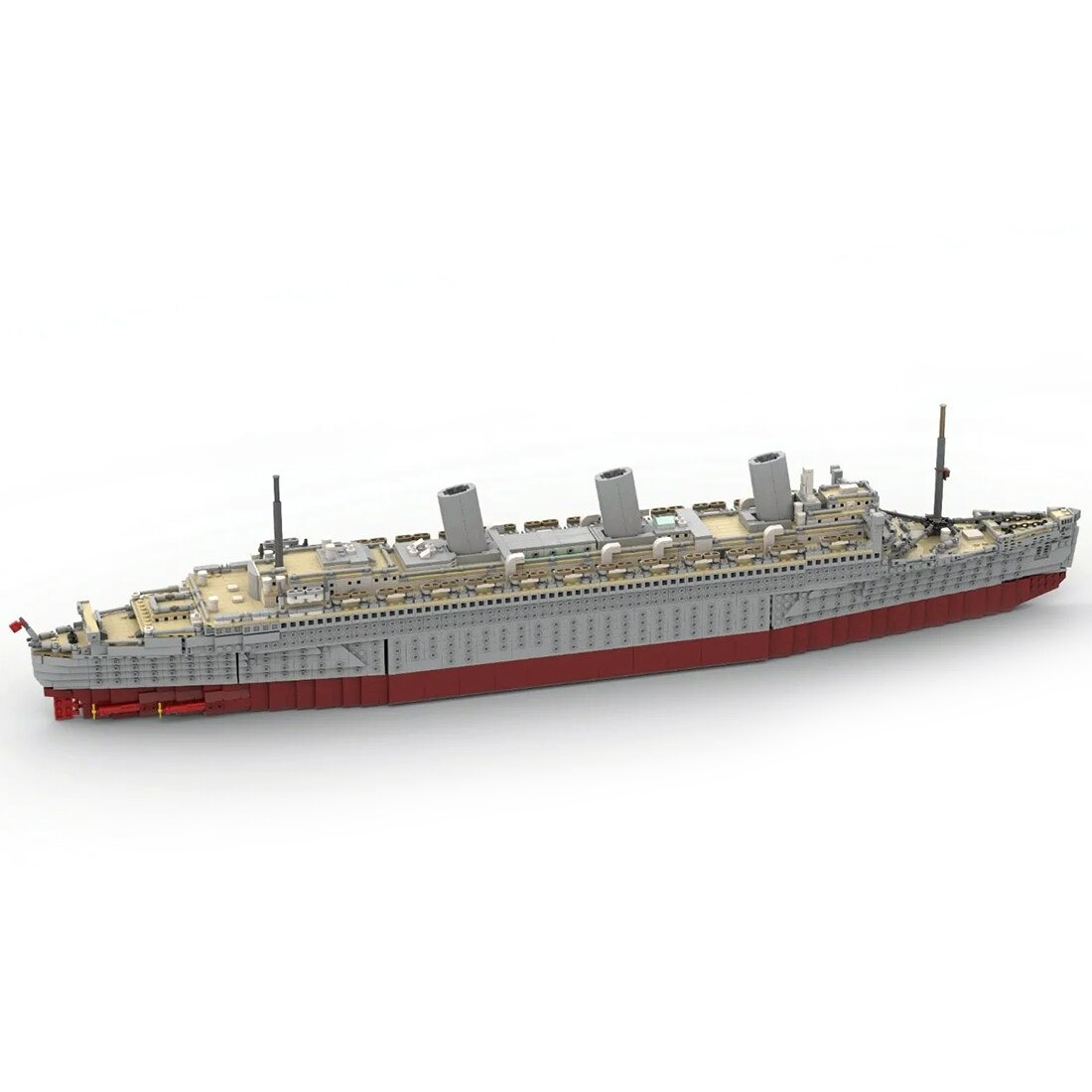This image showcases a detailed model of an ocean miner ship. The ship exhibits a white and gray structure with a red bottom extending along the entire hull. It features three gray smokestacks positioned in the center, providing an outlet for steam. A long vertical pole stands prominently on the right side of the boat, while the bow is adorned with side-by-side chains, adding to its intricate design. The upper section is adorned with numerous windows, suggesting ample passenger or crew space, though it is not designed as a cruise ship. A red flag waves from the aft end, and small yellow propellers are visible at the stern. The overall composition of the ship suggests a function potentially linked to military purposes rather than commercial cruising. The background is simply white, emphasizing the model's intricate details.